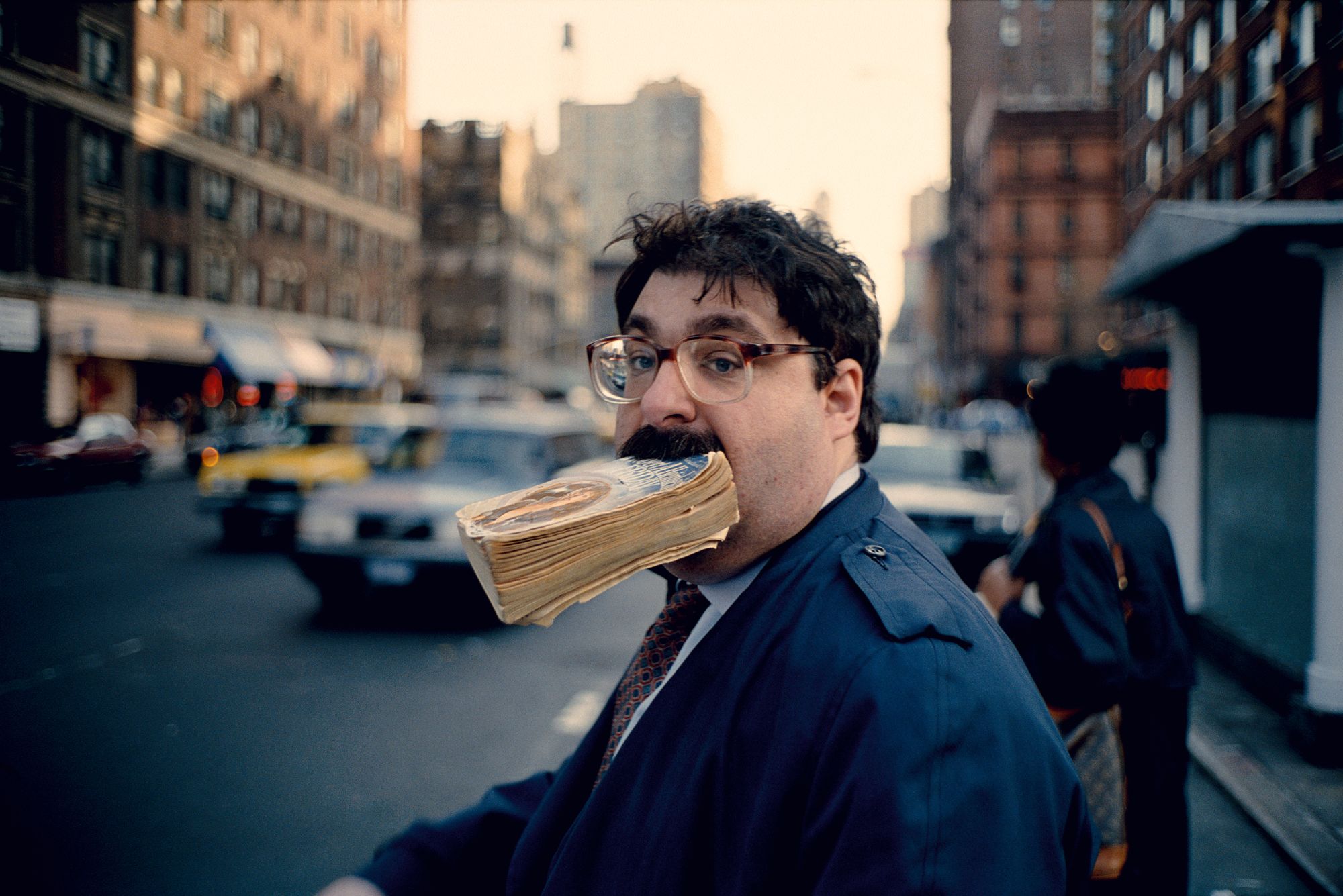The full-color photograph captures a bustling city scene taken outdoors during the day, using natural light. Though it appears unseasonably mild, the mid-to-late autumn or early spring weather is suggested by the attire of the individuals in the frame. The background on the top center consists solely of an expansive, almost empty sky with out-of-focus buildings. Both sides of the image are lined with multi-story brown buildings, hinting at a large metropolitan city, perhaps a downtown area with hints of skyscrapers and shops with awnings.

In the foreground, front and center, stands a heavyset gentleman of Caucasian European descent. He sports slightly messy black hair, tortoiseshell plastic-framed glasses, and a black mustache. His attire includes a dark brown overcoat, a white button-up shirt, and a distinctive blue and red-spotted tie, though some descriptions suggest an orange and black pattern. Notably, he's holding a thick, two to three hundred-page softcover book in his mouth, gripping it with his hands to steady it.

To the lower right, a woman of African descent is captured walking away from the camera. She wears a long dark coat and carries a Louis Vuitton handbag, her black hair visible from behind. In the background towards the left and fading into the center, several cars, including a yellow taxi, a gray car, and a red car, populate the street, all out of focus, enhancing the sense of a lively urban environment. The combination of these elements conveys an intricate and vivid snapshot of an everyday city life moment.